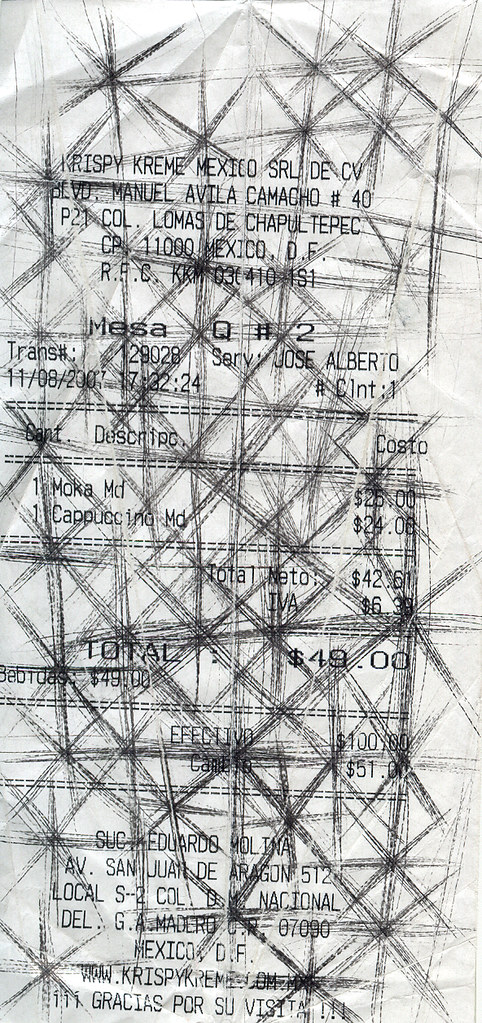The image depicts a white shopping receipt with black printed text, issued by Crispy Cream Mexico SRL DE CV. The top of the receipt prominently displays the business name "Crispy Cream Mexico SRL DE CV," followed by additional information in Spanish, which is partially obscured. The visibility is compromised as thick, crisscrossing diagonal lines have been drawn over the text with a pencil, making parts of the receipt difficult to read.

Below the business name, the address reads, "Manuel Avila Camacho No. 40 P21," located in "COL Lomas de Chapultepec, CP 11000, Mexico DE F RFC." Further down, there is another line mentioning "Mesa Q No. 2." The receipt lists items such as one "Mocha MD" and one "Cappuccino MD," priced at 24.08 pesos and 25 pesos respectively. The subtotal amounts to 42 pesos and some additional cents. The total, with what appears to be a tip included, sums up to 49 pesos. The receipt contains typical Spanish text one might find on a standard commercial transaction receipt.